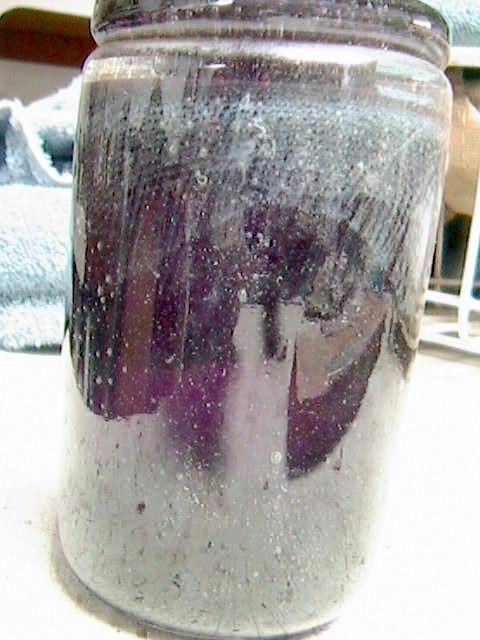In this close-up image, a central jar prominently occupies the scene, set against a whitish background and resting on what appears to be a desk. The jar is crafted from a white clay material adorned with intricate purple designs, suggesting a handmade pottery piece with painting marks indicating encapsulation. The jar's exterior appears somewhat dirty, but inside, it contains layers of substances that give it a colorful and textured appearance. The bottom layer is a light-colored sand, transitioning to a darker purple sand higher up, and then becoming lighter again toward the top. The surroundings are slightly out-of-focus, but a blue towel-like rug lies curled on the left, while a brown countertop is visible beneath the various items. On the right, another desk holds an unspecified item, subtly contributing to the composition's balance. The detailed textures and colors within the jar, combined with the simple yet diverse backdrop, create an intriguing and detailed focal point.